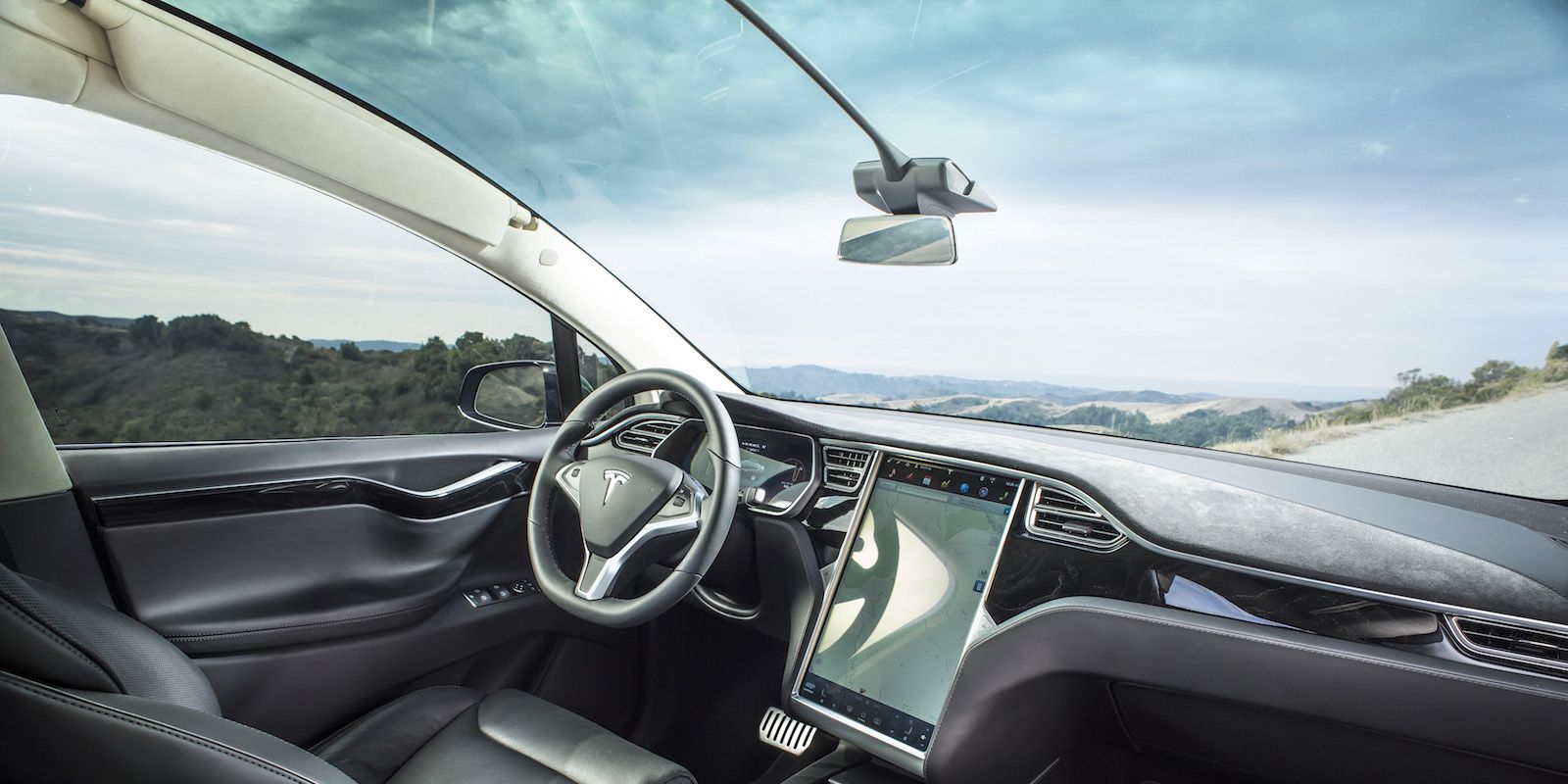This image captures the interior of a sleek Tesla vehicle on a bright, clear day, with vibrant trees and a road visible through the expansive windshield. Dominating the dashboard is a large touchscreen tablet, centrally located and flanked by modern air vents. The dashboard itself presents a sophisticated blend of gray and black hues, complemented by the Tesla logo on the left-side steering wheel. The car’s seats are upholstered in what appears to be premium black leather, adding to the luxurious feel of the interior. Notably, the rearview mirror is centrally positioned at the top of the windshield. The scene outside, showcasing blue skies, undulating hills, trees, and glimpses of winding roads, combines with the car’s detailed interior to create the almost surreal impression of an animated image.